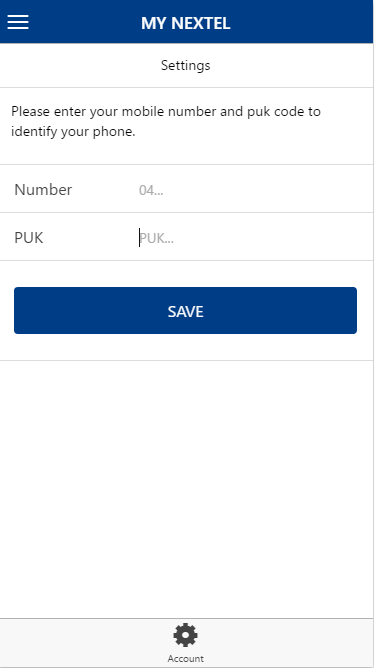This image depicts the login screen of an app, showcasing a user-friendly interface predominantly in blue, white, and black. At the very top, a blue bar spans the width of the screen, featuring white text and a menu icon symbolized by three horizontal lines on the left side. Centered within the blue bar is the bold text "My Next Tell."

Just below this bar, the main section of the screen displays a white background with standard black text. The section is headed by the word "Settings," following which the instruction reads, "Please enter your mobile number and PUK code to identify your phone."

Two clearly defined text boxes are positioned below these instructions. The first text box, labeled "Number" on the left, contains a placeholder gray text starting with "04..." indicating the format of the phone number to be entered. The second text box, labeled "PUK" in capital letters, has a similar placeholder text, "PUK...," where the cursor is already blinking, ready for the user to input their code.

Lower still is a prominent blue button with white text labeled "Save," inviting users to submit their entered details. The bottom portion of the screen consists of some white space, leading down to a section featuring a cog wheel icon typically associated with settings. The button next to this cog wheel is marked "Account," potentially providing access to account-related options.

In summary, the interface is clean, intuitive, and geared towards ensuring users can easily input their necessary information and navigate the app settings.